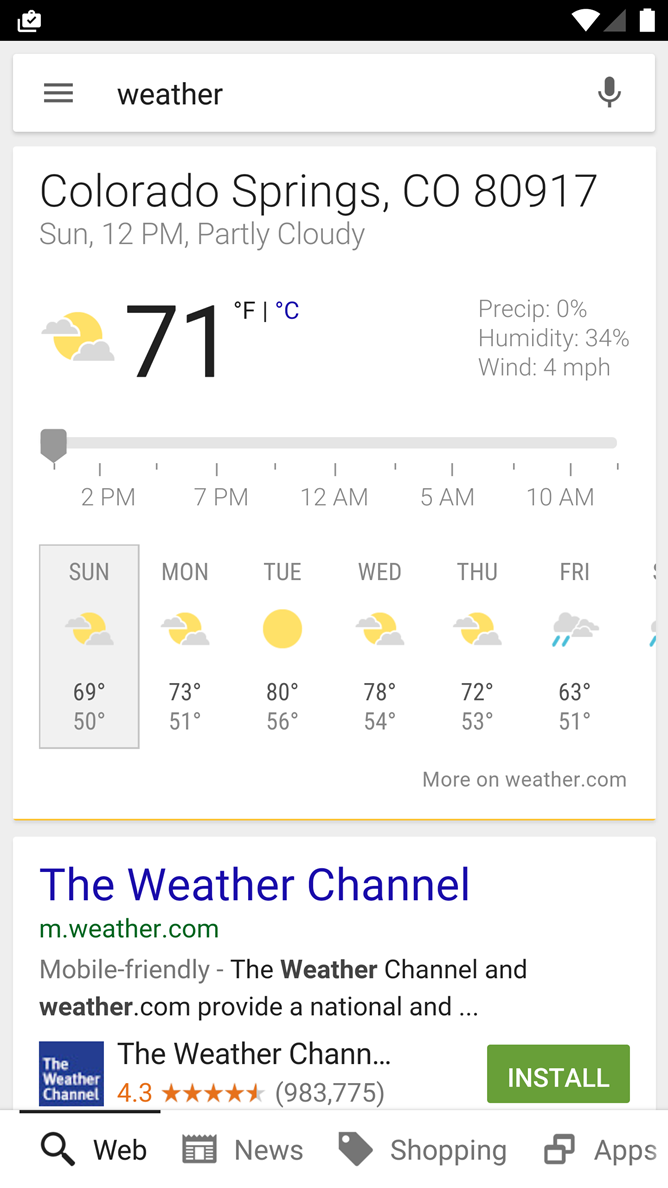The image features a weather application interface, rich with detailed information. 

In the top left corner, there are icons of suitcases with a check mark, potentially indicating a saved or searched location. On the top right, the Wi-Fi icon is fully illuminated, while the service indicators are empty, and the battery icon shows full charge. Below these icons is a hamburger menu icon, suggesting the presence of customizable options or additional settings.

Prominently displayed below these elements is a heading that reads "Weather." Adjacent to it on the right is a microphone icon, possibly for voice search functionality.

Taking center stage is a large information box showing the weather for Colorado Springs, Colorado, 80917. The current conditions are noted as "sunny" at 12 p.m. with a partly cloudy sky graphic, indicating a temperature of 71°F (with a blue icon for Celsius conversion). Additional data points include 0% precipitation, 34% humidity, and 4 miles per hour wind speed.

Below this is a slider bar which can be adjusted to show weather forecasts from 1:30 p.m. to 10:30 a.m. over the next period, though the range appears somewhat unusual.

The forecast for the upcoming days is detailed in a weekly overview:
- **Sunday:** Partly cloudy, high of 69°F, low of 50°F
- **Monday:** Partly cloudy, high of 73°F, low of 51°F
- **Tuesday:** Sunny, high of 80°F, low of 56°F
- **Wednesday:** Partly cloudy, high of 78°F, low of 54°F
- **Thursday:** Partly cloudy, high of 72°F, low of 53°F
- **Friday:** Rain, high of 63°F, low of 51°F

At the bottom, a link to The Weather Channel's mobile site (m.weather.com) is provided, with a note that more detailed information can be found there. To the left of this link is The Weather Channel logo, showing a rating of 4.3 stars out of 5 from 983,775 reviews, with a green "Install" button beside it. Below the main interface, there are tabs indicating additional content categories such as Web, News, Shopping, and Apps.